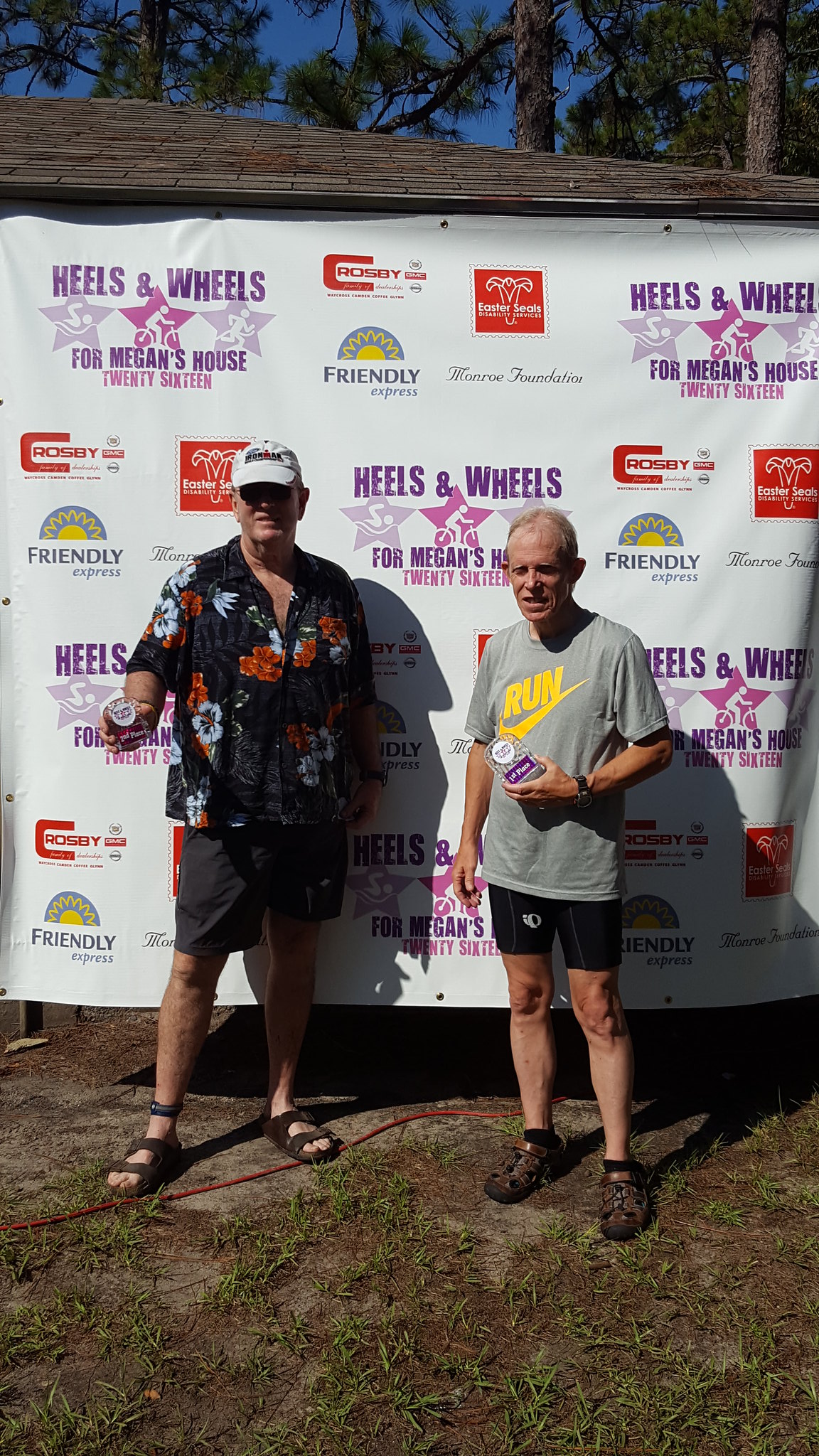In the vertically aligned rectangular picture taken at a sporting event, two men are prominently featured standing in front of a large banner hung from a building. The banner, white with multiple repeated words in purple, reads "Heels and Wheels for Megan's House 2016" and lists sponsors such as Friendly Express, Monroe Foundation, and Crosby. The ground beneath the men is a mixture of dirt and grass, with a red extension cord running between them.

The man on the left, who is slightly heavyset, is dressed in a black, orange, and white floral shirt with the first couple of buttons unbuttoned, a white ball cap with writing on it, black shorts, and brown sandals. He is also wearing sunglasses. The slender man on the right is dressed in a gray Nike t-shirt that says "Run" with a yellow Nike symbol, black shorts, and sandals that appear to be Crocs. He has gray hair and is not wearing a hat. Both men are holding objects in their hands, seemingly related to the Wimbledon logo. They appear to be supporting or have participated in a race linked to the event advertised on the banner behind them.